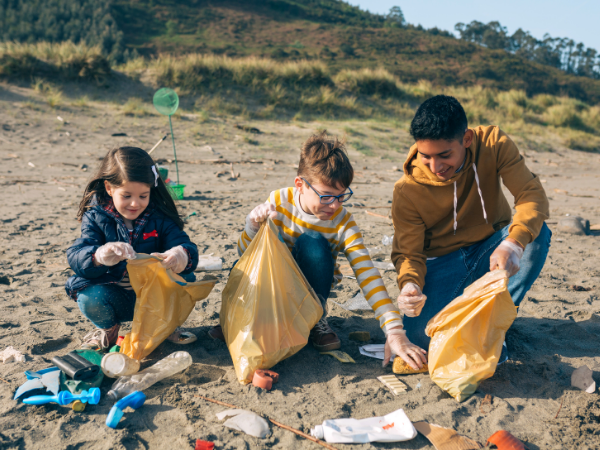In this detailed vertical rectangular outdoor image, three children are diligently cleaning up a trash-strewn beach under a clear blue sky visible in the corner. The scene is set in front of a small hill covered with dry, brown grass. Dispersed across the brown sand are various pieces of trash, including colorful pieces of paper and plastic bottles in shades of blue, white, and red.

The children are equipped with yellow plastic bags, which are semi-transparent, and are wearing white plastic gloves as they work together to clear the litter. On the left is a little girl with long dark brown hair, adorned with a bow, wearing a blue jacket over a blue and white striped shirt and blue jeans. She is crouched down, intently picking up trash. 

Next to her in the middle is a young boy with brown hair and glasses, dressed in an orange and white striped shirt, tan shoes, and jeans. He is also picking up trash, though in some descriptions, it appears he may not be wearing gloves.

On the right is an older boy, possibly Hispanic, characterized by his dark hair and skin. He is wearing a dark yellow pullover hoodie with blue pants and is engaged in the cleanup effort alongside the other two children. The shared emphasis among the contributors highlights the coordinated cleanliness effort and the children's collaborative spirit in restoring the beauty of the beach.